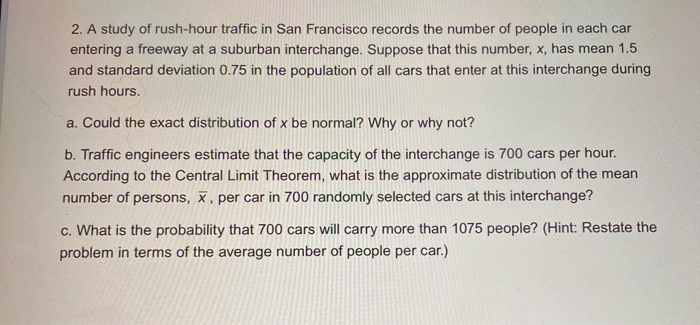The image depicts a screen capture of a computer screen displaying a paragraph of text on an off-white background. The black text appears to be part of a typed mathematics or statistics question set focused on rush hour traffic in San Francisco. It starts with "2." and discusses a study that records the number of people in each car entering a freeway at a suburban interchange. The variable \(X\) has a mean of 1.5 and a standard deviation of 0.75 for the population of all cars entering at the interchange during rush hours.

The first part, labeled "A," asks, "Could the exact distribution of \(X\) be normal? Why or why not?" The second part, labeled "B," states that traffic engineers estimate the interchange's capacity at 700 cars per hour, and questions the approximate distribution of the mean number of people, \( \overline{X} \), per car in 700 randomly selected cars, according to the central limit theorem. The final part, labeled "C," inquires about the probability that 700 cars will carry more than 1,075 people, with a hint suggesting to restate the problem in terms of the average number of people per car. The entire text is clear, and the image shows fine pixelation indicative of a picture taken of a computer screen.